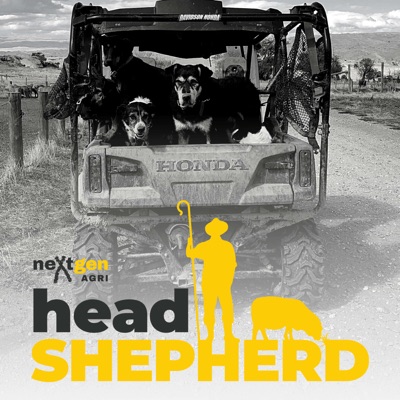The black and white, square-shaped advertisement depicts a Honda utility vehicle parked on a gravel road beside a large pasture and wooden fence posts. The vehicle, which is a cross between a truck and an ATV, features an open bed in the back where two prominent dogs with white-marked faces and floppy ears stand alert, staring directly at the viewer. One dog is black and tan while the other is tricolored. A partly cloudy sky serves as the backdrop, emphasizing the rural setting with its expansive fields and scattered trees. At the bottom of the image, the text "Next Gen Agri" is displayed, with "Next" and "Agri" in black and "Gen" in yellow, where the "X" stylized to resemble sheep shears. Below it, the text "HEAD SHEPHERD" appears, where "HEAD" is in dark gray and "SHEPHERD" in bold yellow, accompanied by a yellow silhouette of a man holding a shepherd's hook with a sheep beside him.